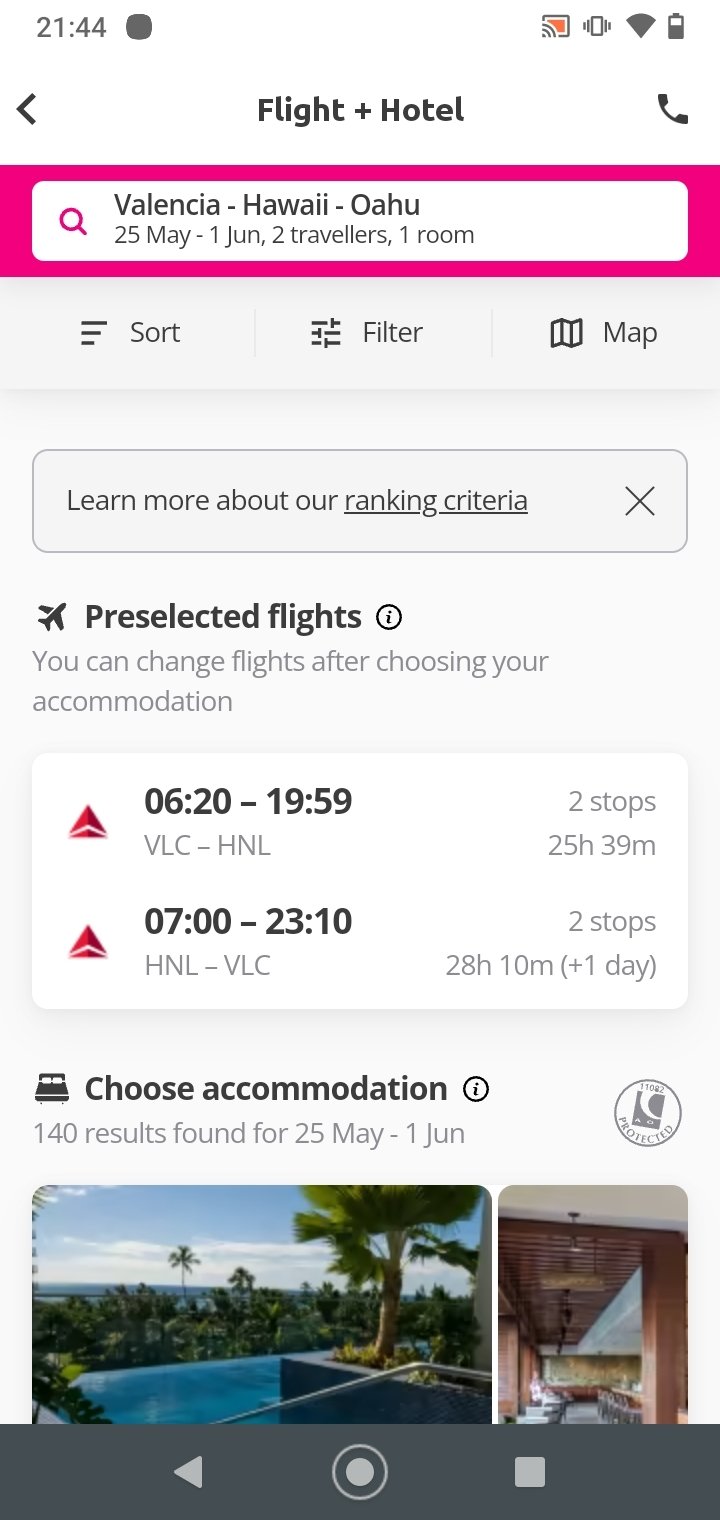A phone screen displays a travel search for flights and hotels. At the top, there is a white bar containing the time in black text on a black square, a half-full battery icon, and full Wi-Fi signal with the phone on vibrate mode. Below this, a black bordered area with orange highlights has a phone icon in the center and the bolded text "Flight + Hotel." To the left, there is a greater than sign pointing left, next to a pink triangle containing a white search bar. The search bar features a pink search icon on the left with bold black text reading "Valencia - Hawaii - Oahu." Beneath this, in smaller black text, are the date, number of travelers, and number of rooms.

Further down, black text reads "Sort," "Filter," and "Map," each with icons to their left. Below this, another black-bordered rectangle contains the underlined text "Learn more about our ranking criteria" with a black 'X' on the right. Beneath this section is an airplane icon, followed by bold black text stating "Pre-selected flights" alongside a white circle with a black border and a black lowercase 'i' inside. Two lines of flight information are provided underneath.

In a white rectangle below, two airlines are listed with their emblems on the left, followed by departure times and locations, and details on the number of stops and total travel time on the right. Below this information, black text reads "Choose accommodation," with a bed icon next to it. At the bottom, black text states "140 results found for 25 May - 1 June." The screen also shows two images: one of an outdoor pool with trees and sky, and another of a room's interior.